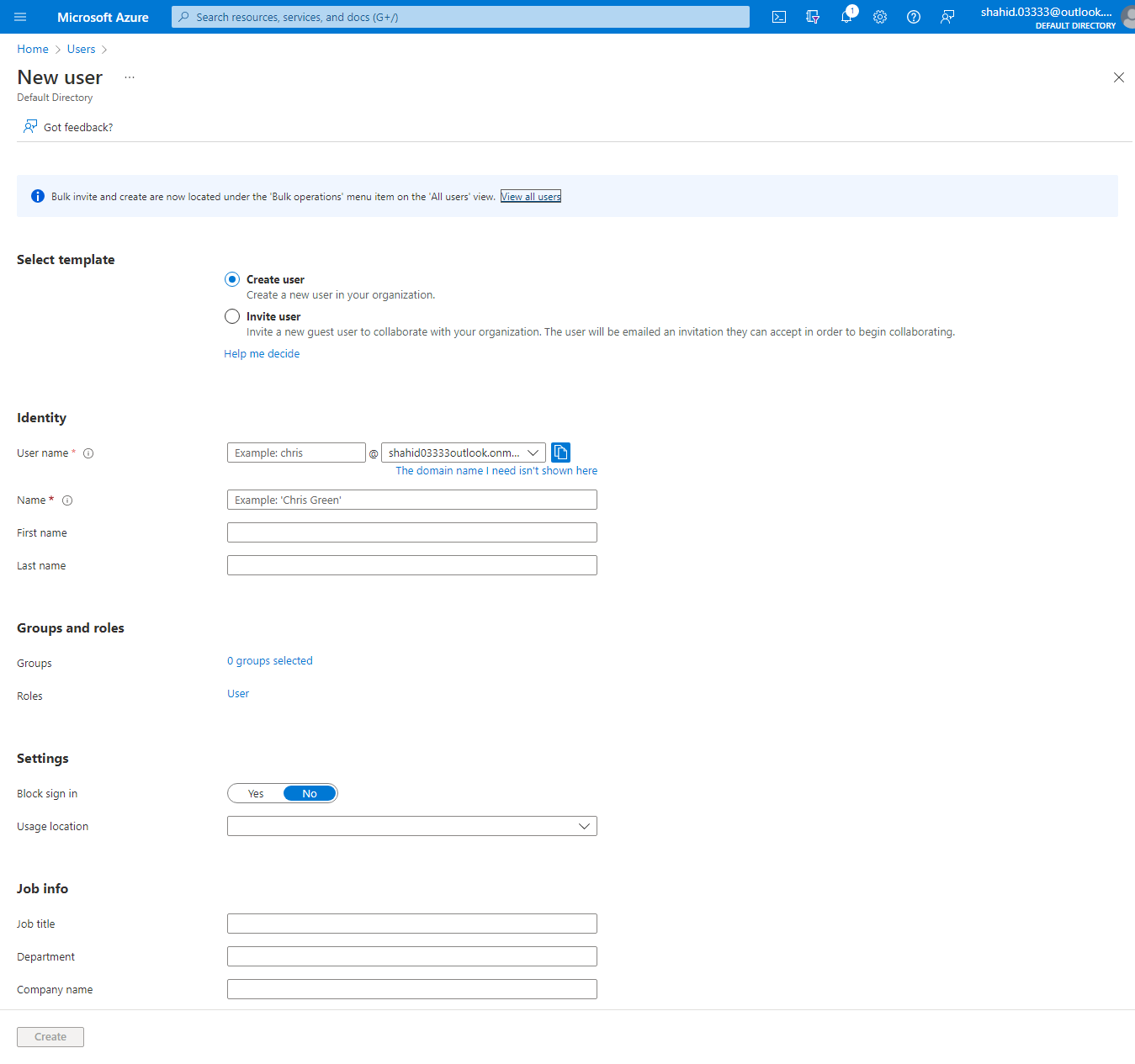This image showcases a Microsoft Azure web page interface. Prominently displayed at the top center is a search field labeled "Search resources, services, and docs." The top navigation bar includes options such as Home and Users. A new user interface message indicates that "Bulk invites and creates are now located under the bulk operations menu." 

In the main section of the page, there is a detailed view titled "All Users," which allows the user to see and manage various user profiles. The top right corner of the page displays the username "Shahid.0303333," logged in currently. 

On the top left, shortcuts to other Microsoft services, such as Outlook, are visible. Detailed user information fields are listed, including identity, username, name, first name, last name, groups and roles, settings, blog sign-in, usage location, job title, department, and company name. The primary colors used in this interface are blue, white, and black, adhering to Microsoft's typical branding.